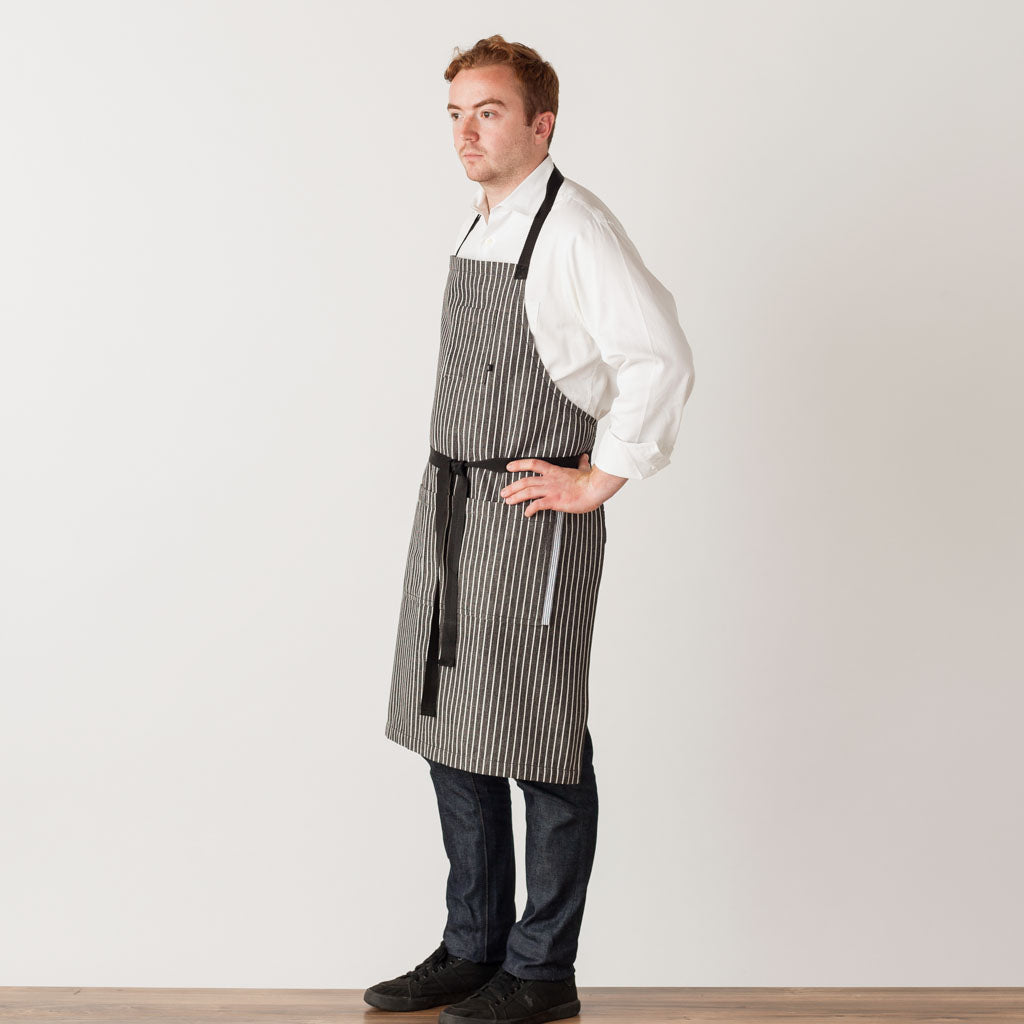This image features a man dressed in what appears to be a cook's uniform. He is positioned against a very light, medium-light gray wall with a brown, medium-wood floor beneath him. The man is standing in a three-quarters profile, looking towards the left with a concerned expression on his face. He is attired in a white button-up shirt, open at the collar and rolled up slightly above the wrists. Over his shirt, he wears a black and white striped apron that has a black neck strap and is tied in the front with a black tie around his waist. The apron also has pockets. He is wearing dark blue jeans and black shoes, possibly sneakers. His left hand is placed on his hip, which is the side facing the camera. The man has short, wavy reddish-brown hair, styled longer on the top and curving to his right, with matching colored eyebrows, brown eyes, and a slight outline of a mustache along with a bit of stubble.